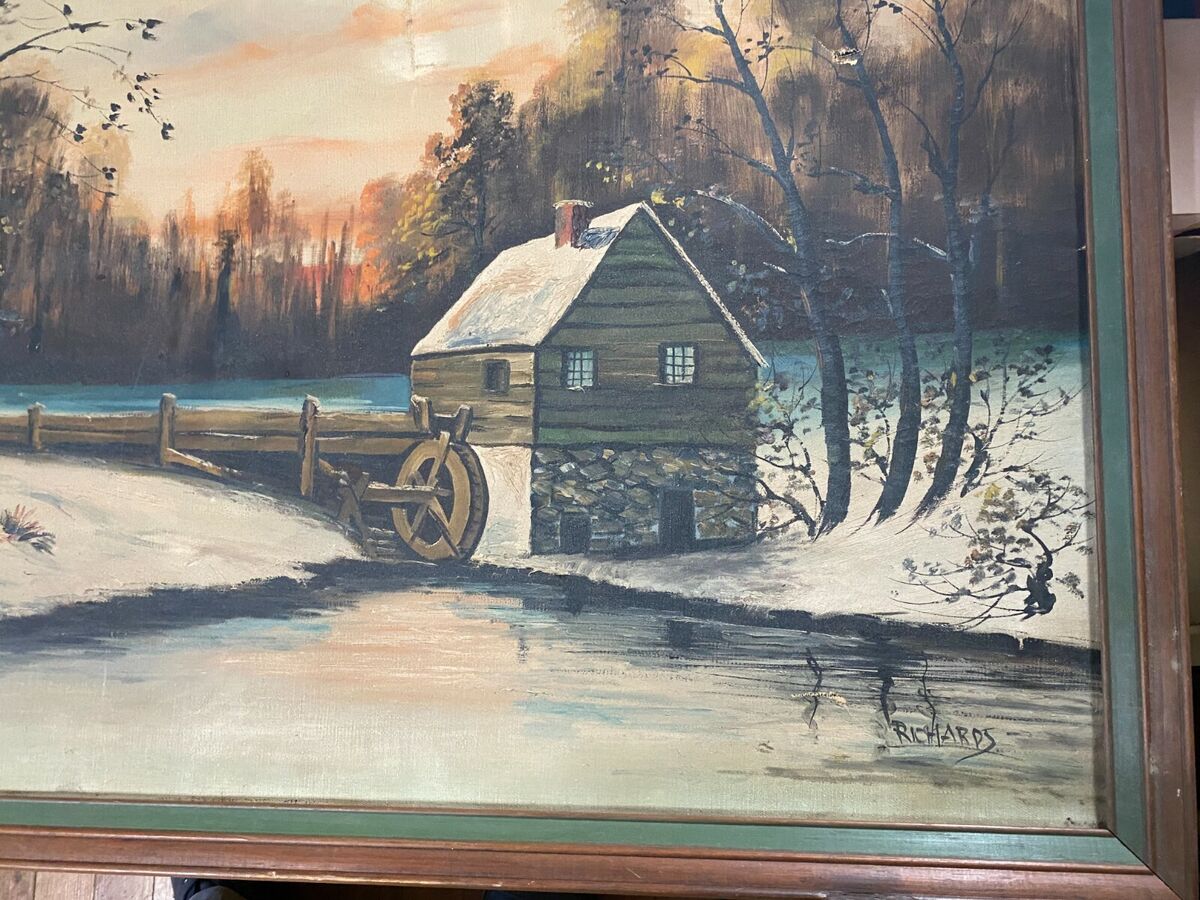This is an intricately detailed drawing of an old stone and wood mill during a winter sunset, signed by Richards in black in the lower right-hand corner. The structure consists of a stone masonry base supporting an upper wooden living area, capped by a white roof blanketed in snow. A small red chimney protrudes from the roof. Prominently, a large water wheel stands beside the house, indicating its historical function as a mill. A wooden bridge spans a broad creek, narrowing as it approaches the wheel to maximize its power. The water in the creek displays an array of peach, blue, and white tones, reflecting the sky's cream, orange, and blue hues. Trees, both near the mill and in the distance, border the scene, their bare branches silhouetted against the vibrant sky. Snow covers the ground, and the scene is framed by an elegant brown border, enhancing its rustic charm.